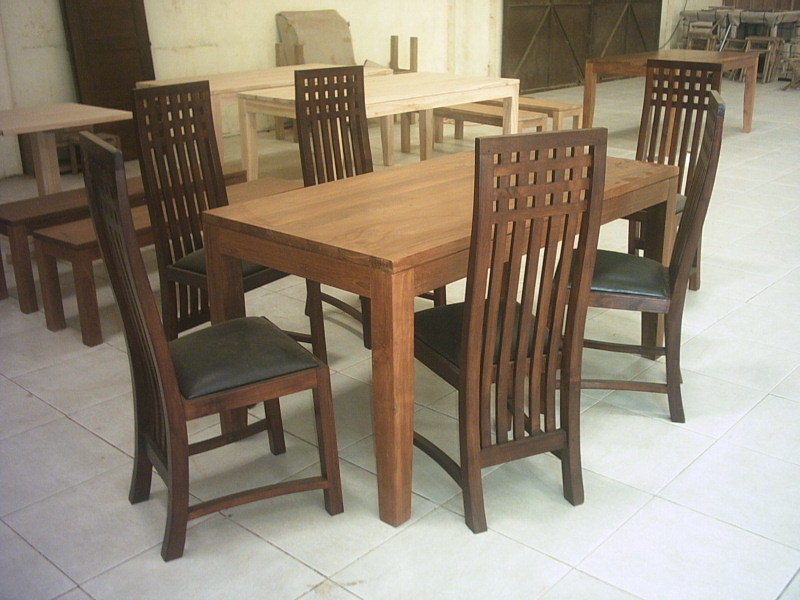This photograph, possibly taken in a furniture workshop or warehouse, captures a rectangular wooden dining table with a light to medium brown finish and a strong wood grain. The table, supported by four sturdy legs, is surrounded by six dark brown wooden chairs. Each chair features a distinct design with a very long, slightly curved back comprised of vertical and horizontal timber planks that extend down to a cross beam on its legs. Additionally, the chairs are topped with black padded cushions for comfort. Arranged symmetrically, two chairs are positioned at each length of the table, and one at each end. 

In the background, several other tables can be seen, some of which appear to be in various stages of completion, suggestive of a furniture manufacturing or storage environment. There are lighter wood tables and brown benches, as well as additional furniture items stacked or displayed along a white concrete wall. A distinctive, large double-wide barn door with supporting struts is visible, alongside what seems to be a darkly stained wooden door leaning against the wall. The room has a floor made of white square tiles, approximately 20 inches in size, reinforcing the industrial or warehouse setting.